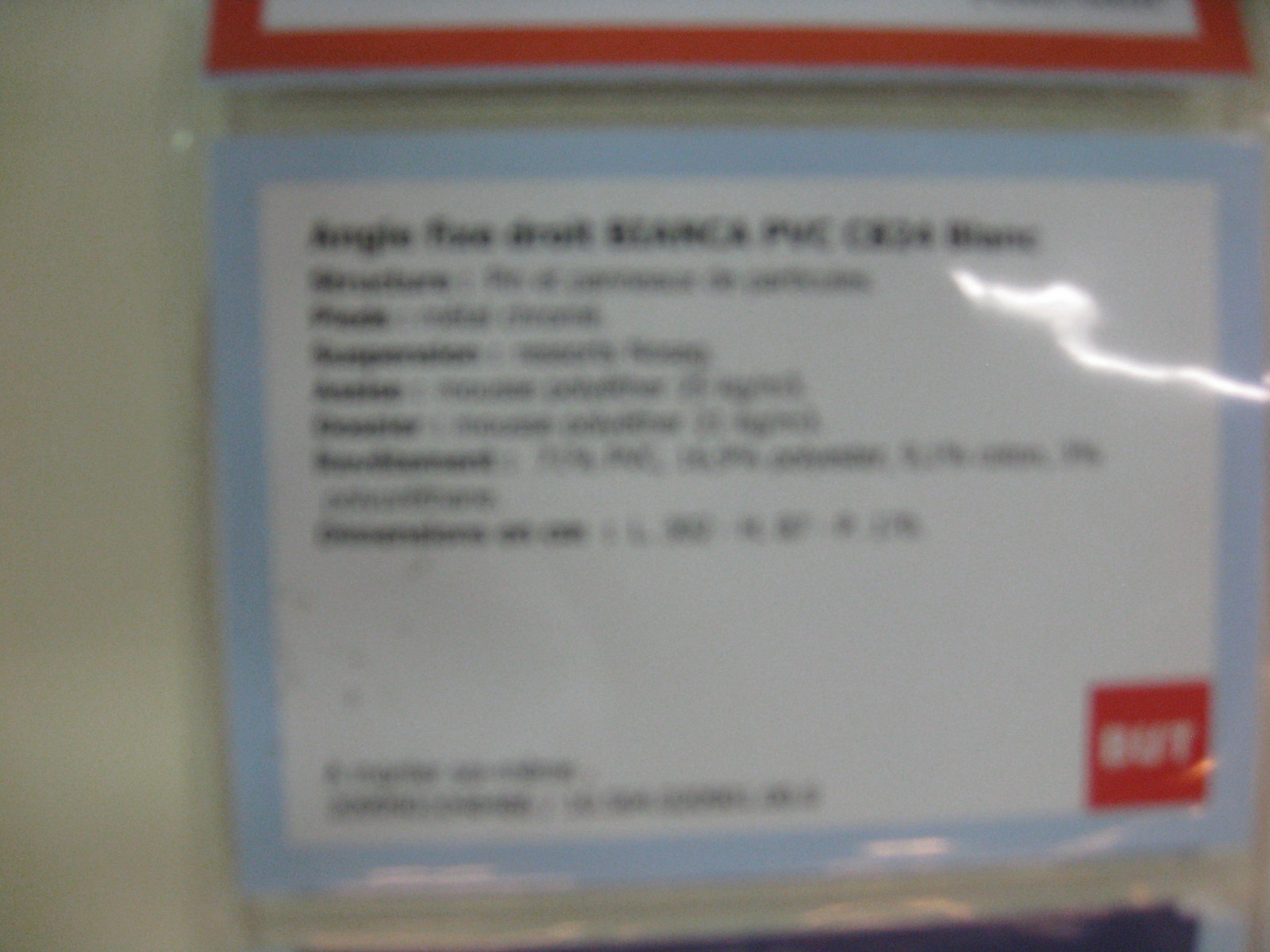This image depicts a blurry, low-resolution, square-shaped photo primarily featuring a card that nearly occupies the entire frame. The card itself is also square, outlined with a light blue border. In the bottom right corner of the card, there is a small red square. The central background of the card is white, and although there is black text in the middle, the image's poor quality makes the text illegible.